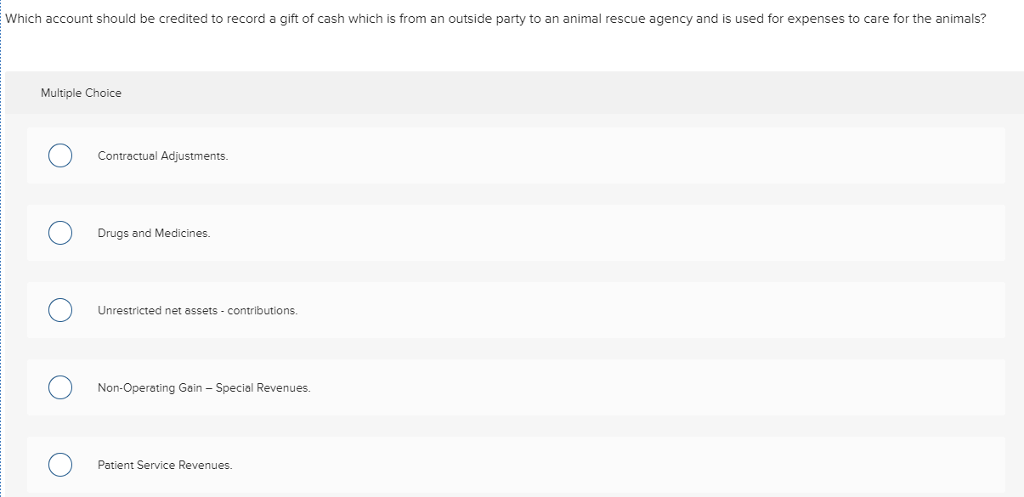The image depicts a multiple-choice question layout commonly used in quizzes or exams. There are several different sections, each represented by white and gray rectangles with text inside. 

At the very top, there is a white rectangle containing black text that reads: "Which account should be credited to record a gift of cash from an outside party to an animal rescue agency, used for expenses to care for the animals?" 

Below the question, there is a darker gray rectangle that indicates: "Multiple Choice."

Following this are five light gray rectangles, listed vertically from top to bottom. Each rectangle has a corresponding blue-outlined circle, suggesting that these are options for a multiple-choice question where the user should mark one circle.

The five options are as follows:
1. "Contractual Adjustments"
2. "Drugs and Medicine"
3. "Unrestricted Net Assets Contributions"
4. "Non-Operating Gain Special Revenues"
5. "Patient Service Revenues"